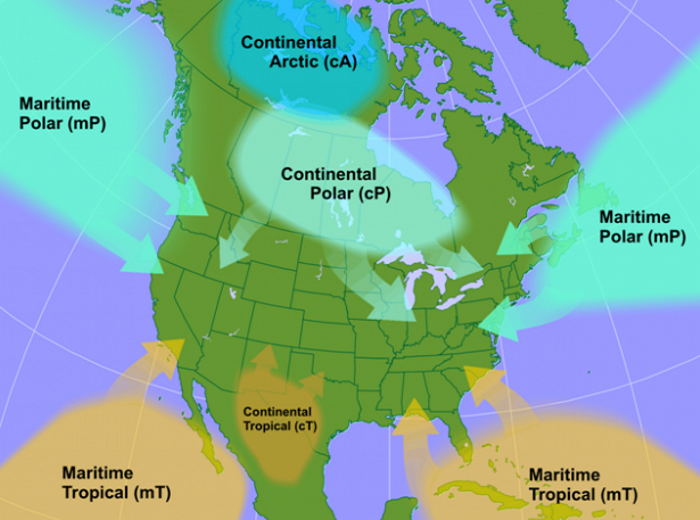This detailed illustration in landscape orientation presents a color map of North America, including the continental United States, Canada, Greenland, Mexico, and parts of Central America. The landmasses are depicted in a dark green hue, set against surrounding waters colored in light purple. The map is overlaid with several pastel-colored conversation clouds, each labeled with descriptions of different air masses in black text. Starting from the top and moving clockwise, the labels read: Continental Arctic (CA), Continental Polar (CP), Maritime Polar (MP), Maritime Tropical (MT), and again Maritime Tropical (MT) and Maritime Polar (MP) at the lower left and top left respectively. The map also shows various arrows illustrating the flow and influence of these air masses, indicating seasonal weather patterns. Identifiable regions include Maritime Polar air descending into Washington and Oregon, Continental Arctic and Polar air at the top, Maritime Polar air off the Atlantic Ocean, Maritime Tropical air on the lower right and left, and Continental Tropical air over Texas. This graphic design and text-based map provides an engaging, visual representation of the climatic conditions affecting North America.